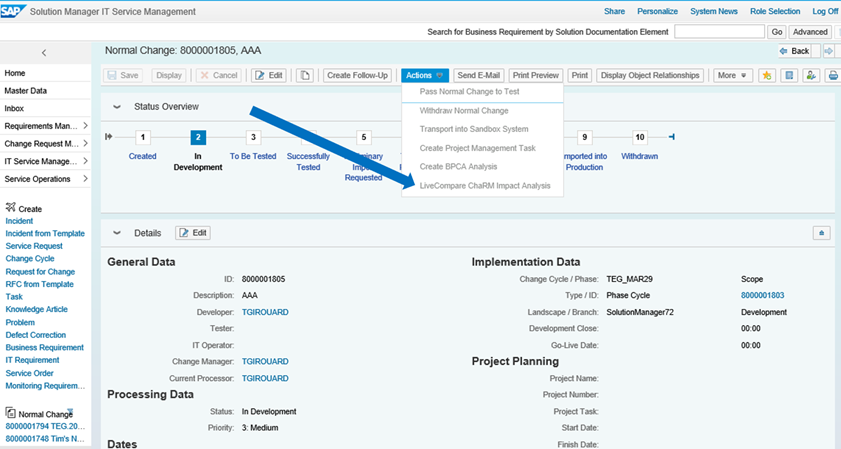This detailed descriptive caption is for a screenshot from a software application window.

---

In this screenshot from a SAP application, a large blue arrow points to the "Live Compare CHAR-RM Impact Analysis" option within the "Actions" drop-down menu. The application running is the "Solutions Manager IT Service Management" module, evident from the title bar at the top next to the SAP icon. 

On the left-hand side, a navigation menu lists various sections such as Home, Master Data, Inbox, Requirements Manager, Change Request Manager, IT Service Manager, and Service Operations, among other options. This menu allows users to navigate and create different service tasks and tickets.

The main window displays an existing task or ticket, detailing its status and other technical information. The interface features a color scheme dominated by shades of grey and blue, lending a professional and organized aesthetic.